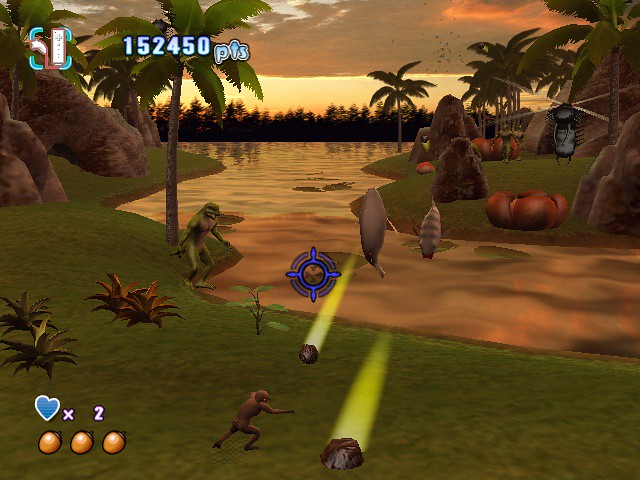The image appears to be a screenshot from a surreal or fantastical video game environment. In the foreground, there are a couple of bright yellow lights illuminating the scene, casting an ethereal glow over the landscape. The scene includes recognizable elements such as palm trees and a gently flowing stream, which add a touch of natural beauty. However, the setting is peculiar, featuring a mix of bizarre and whimsical objects. 

Notably, there is a figure-like object with a propeller on its head, consisting of four spokes, giving it an unusual, mechanical appearance. Scattered throughout the environment, various rocks add texture to the scene. In an extraordinary twist, there appear to be fish moving upright on their tails, gliding across the water’s surface, defying normal aquatic behavior.

On the left side of the image, near a palm tree, a faintly human-looking creature is visible with its arms outstretched, seemingly reaching for something or in a state of anticipation. Nearby, spiky objects resembling sea urchins add to the scene's surreal ambiance. Additionally, a monkey-like creature is also present, its appearance blending into the fantastical elements around it. The overall composition of the image creates a striking and otherworldly visual experience.